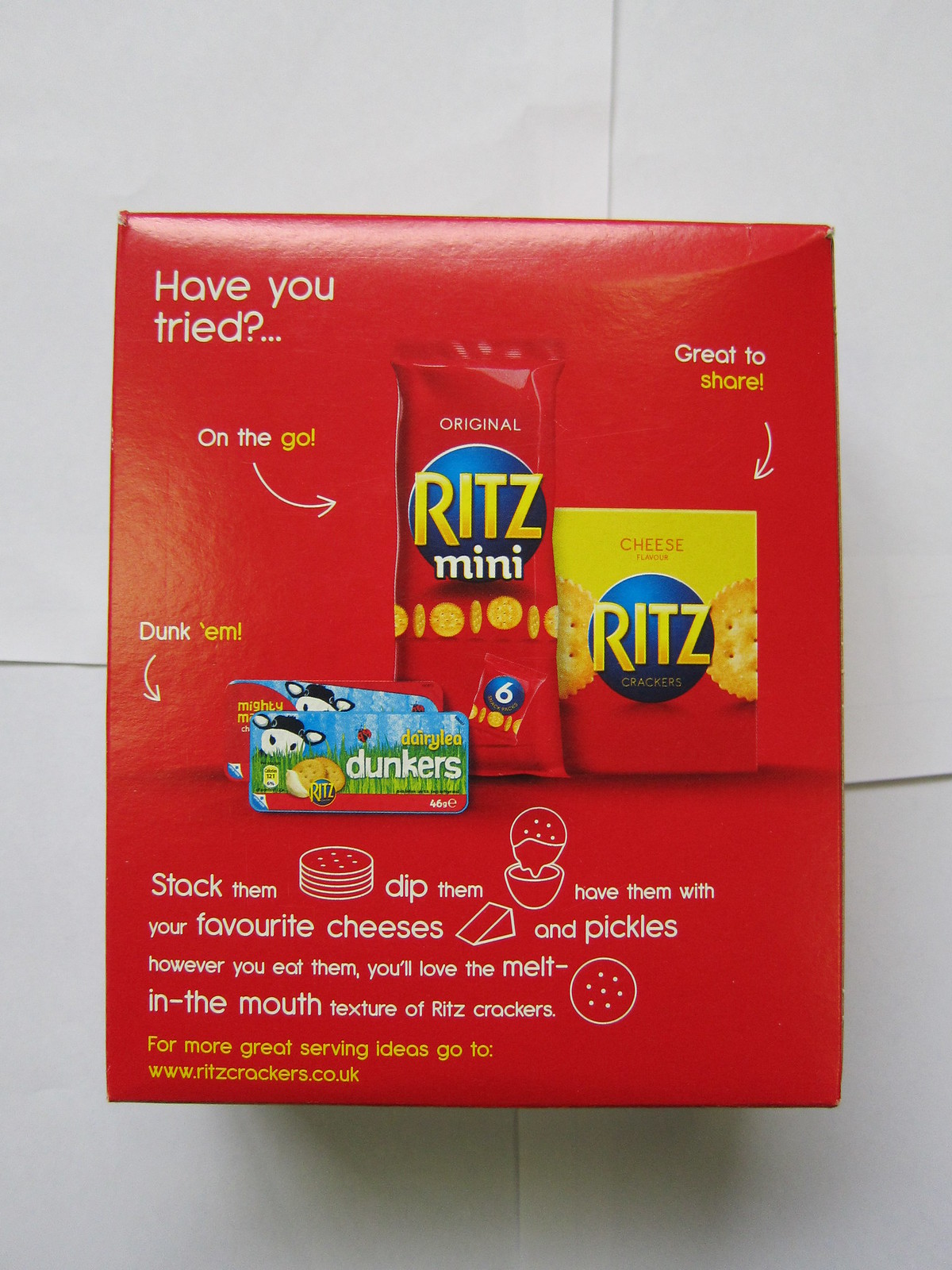The image depicts the back side of a vertical box of Ritz Crackers set against a tile surface. Dominated by the brand's signature red packaging, the top left corner features bold white text reading, "Have you tried?" beneath which an advertisement showcases three different Ritz products. From left to right, there is a red package of Original Ritz Mini labeled "On the go," a yellow and red box of cheese-flavored Ritz Crackers with an arrow pointing to it labeled "Great to share," and Dairy Lee Dunkers by Ritz, highlighted with an arrow that says "Dunk em." Near the bottom section, white text invites consumers to explore various ways to enjoy Ritz Crackers: "Stack them," "Dip them," and "Have them with your favorite cheeses and pickles." It concludes with the promise, "However you eat them, you'll love the melt-in-the-mouth texture of Ritz Crackers," and a call to visit www.ritzcrackers.co.uk for more serving ideas. The color palette in the image includes red, yellow, blue, gray, white, black, and beige.